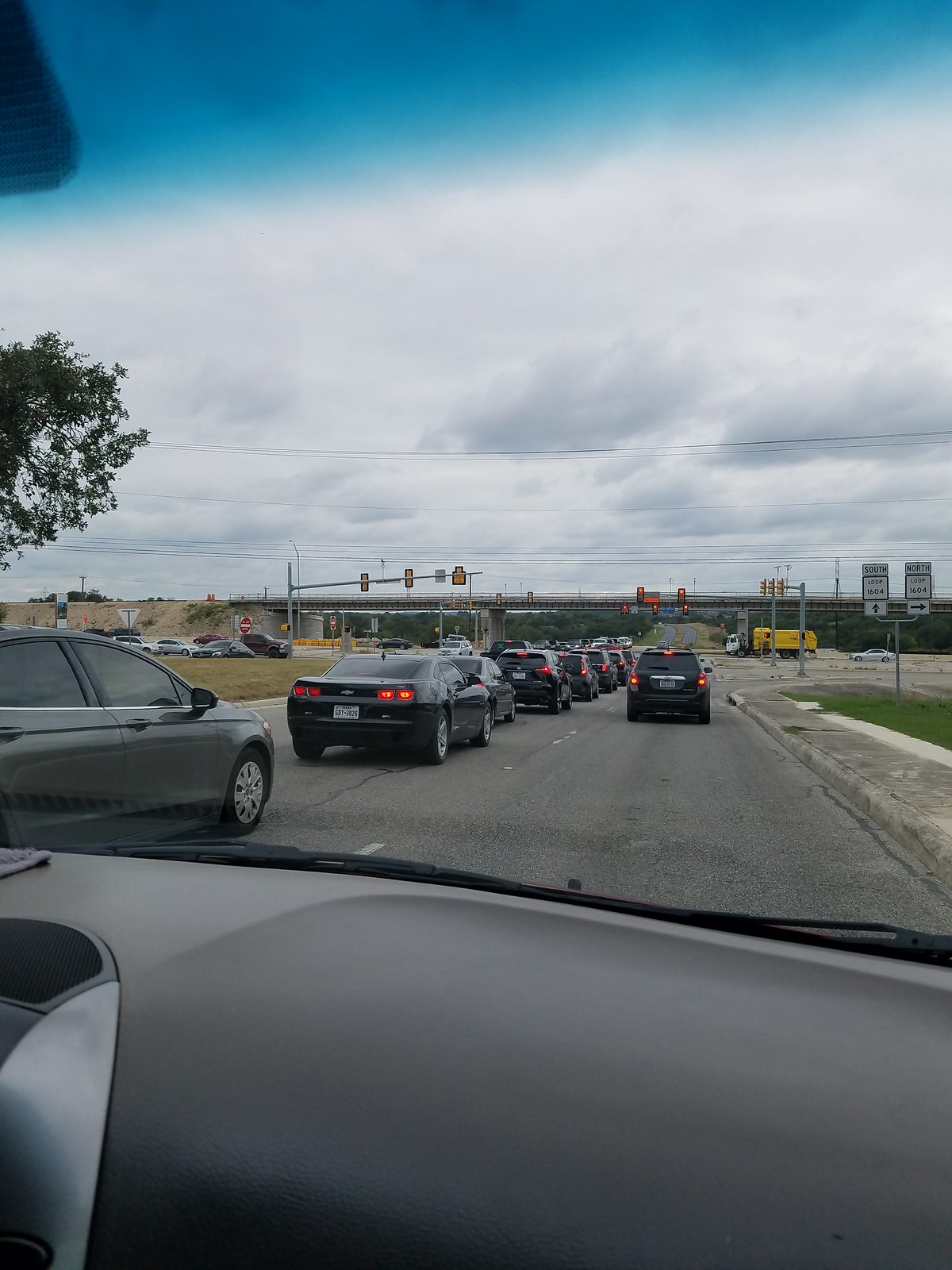The image is captured from the vantage point of the right-hand passenger seat, showcasing a first-person POV from inside a car. The camera is slightly tilted downward, providing a clear view of the dashboard directly ahead. The windscreen's subtle glare and its blue-tinted top edge are evident, highlighting the exterior world beyond. Black windshield wipers are visible at the base of the windscreen. The sky is densely overcast with white clouds, indicating an overcast day. The car is stationary, halted in a line of traffic at what appears to be a red traffic light in the distance. Approximately five to seven meters ahead, a car with illuminated brake lights is visible. To the left, another lane of traffic moves in the same direction, with cars closely packed together without any noticeable gaps.